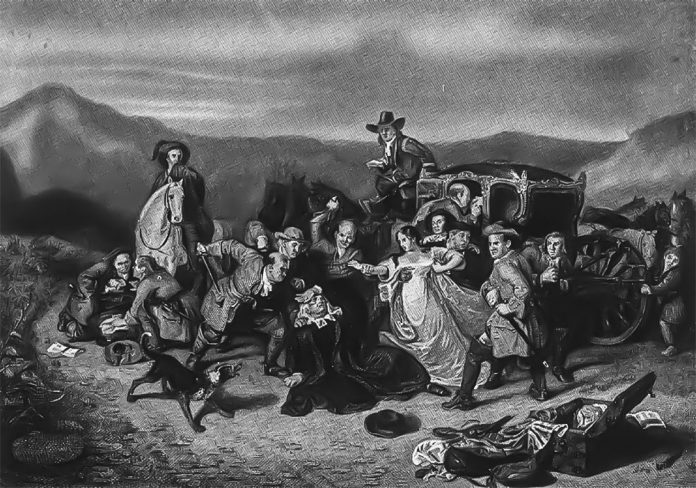The image is a black-and-white representation of what appears to be a historical painting, likely from the 1600s to 1800s. It depicts a chaotic scene on a beaten road with mountains in the background. At the heart of the turmoil, a central figure, possibly a man in a long coat and wide collar, is cowering on the ground with his hands covering his face. Surrounding him are numerous people involved in various aggressive actions. One man stands over the central figure, brandishing a sword, while another appears poised to strike with a raised hand, and yet another readies a dagger. To the right, a woman in a long, flowy dress watches in distress, restrained by two men as she attempts to intervene. A barking dog adds to the commotion, as do the scattered contents of an open suitcase in the lower right corner. A horse-drawn carriage, with people peering through its windows, and another man on horseback wearing a feathered hat, oversees the conflict from the background. In total, there are around sixteen people involved or observing this tumultuous event, all contributing to the sense of urgency and violence in the scene.